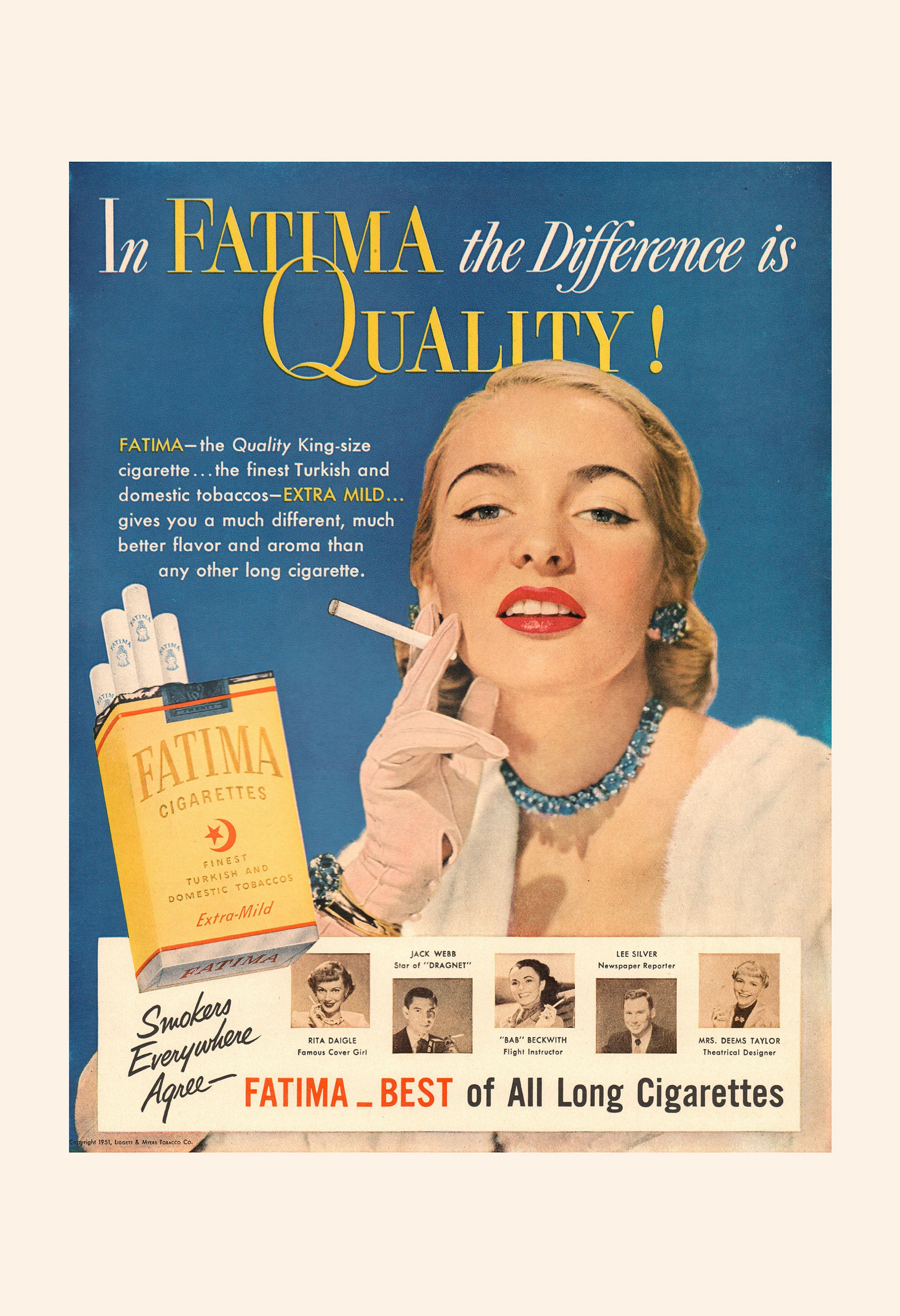This vintage 1950s print advertisement exudes elegance and sophistication in its promotion of Fatima cigarettes. The background is a rich cream color with a prominent blue rectangular section that houses the key elements of the ad. The headline reads "In Fatima, the difference is quality," setting the tone for the luxurious presentation.

At the forefront is an impeccably styled woman with slicked-back blonde hair. She exudes sophistication, smiling directly at the camera while holding a lit cigarette near her cheek with her pink-gloved hand. Her attire includes a white fur-like jacket complemented by a striking blue jeweled necklace and matching earrings.

The advertisement text beside her describes Fatima as "the quality king-size cigarette," made from "the finest Turkish and domestic tobaccos." It promises an "extra mild" experience that delivers a "much different, much better flavor and aroma than any other long cigarette."

To the left of the woman is an image of a gold-colored cigarette pack with the brand name "Fatima" etched in darker gold text. Four cigarettes extend invitingly from the open pack. Below, a white banner displays photographs of five individuals offering testimonials, identified as Rita Daigle, Jack Webb, Bab Beckwith, Lee Silver, and Mrs. Deems Taylor. The slogan underneath encapsulates their collective endorsement: "Smokers everywhere agree, Fatima, best of all long cigarettes."

This advertisement masterfully combines visual appeal with detailed descriptions to emphasize the superior quality and unique experience of smoking Fatima cigarettes.